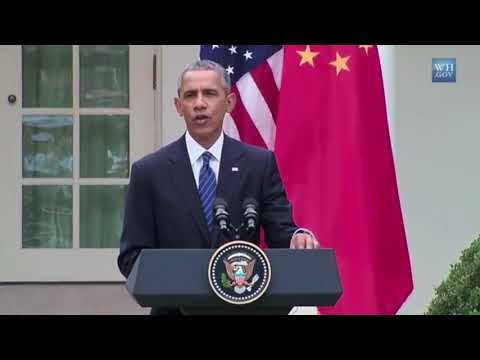This horizontal-rectangular image captures former United States President Barack Obama mid-speech, standing outside, possibly at the White House. Obama is positioned at a black lectern adorned with the presidential seal, which features an eagle encircled by gold stars and framed in gold. The seal rests prominently on the front of the lectern, which also supports two microphones. He is attired in a dark blue suit, complemented by a white shirt and a blue tie with silver accents, and wears a lapel pin.

Behind Obama, to his left, is a white building with a window, and to his right, a door with glass panes reflecting the surroundings. Flanking him are two flags: the American flag and another red flag with gold stars, likely representing China. A green bush peeks into the frame from the top right corner, adding a touch of greenery to the scene. The text "WH.gov" is visible in a blue box in the upper right corner. Obama has a serious expression, with his mouth slightly open as he addresses the audience, conveying a sense of concentration and purpose. The focus of the image spans from his waist upwards, highlighting his presence and composure as he speaks.